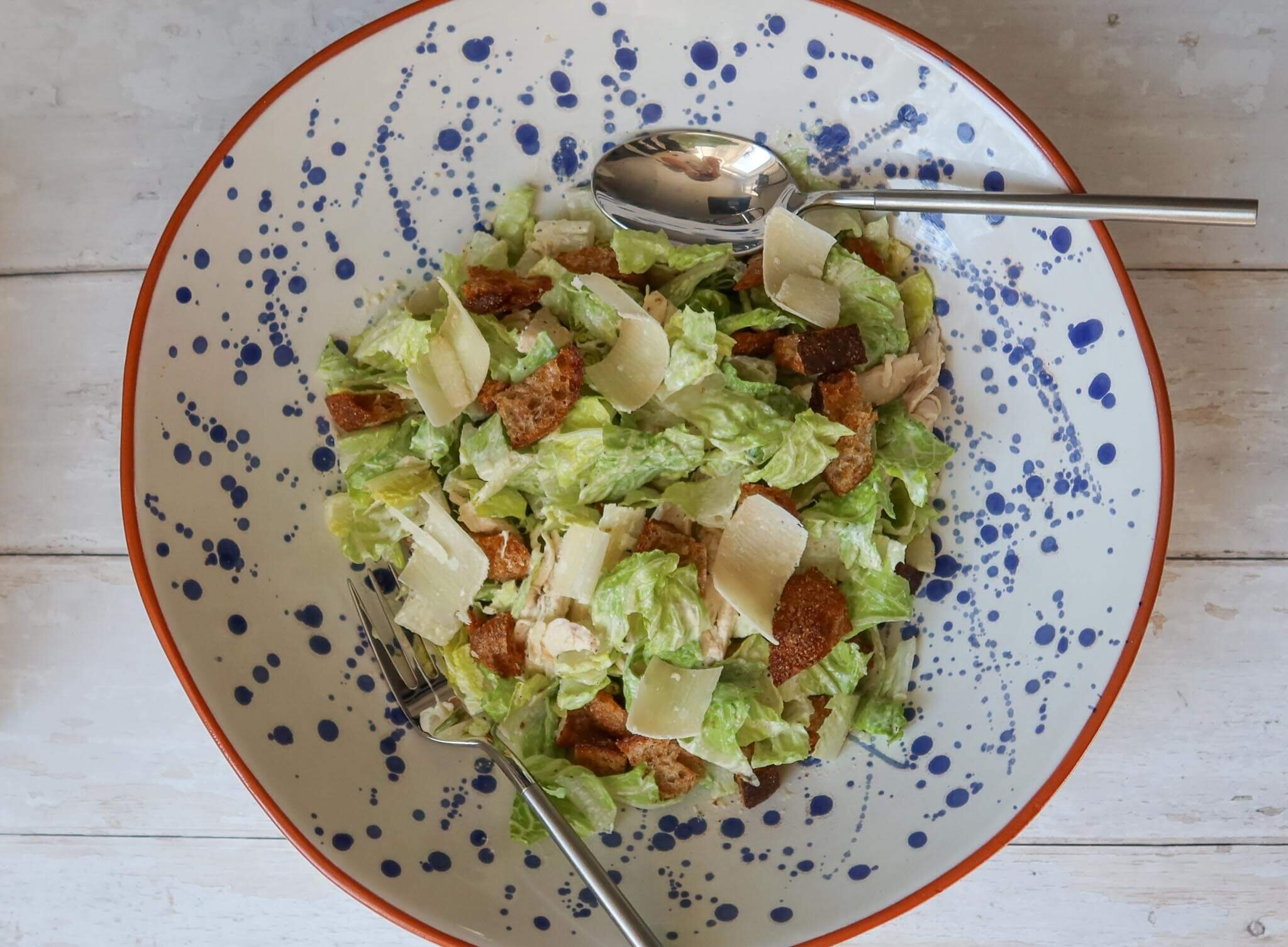This overhead image showcases a rustic, unevenly circular white plate adorned with blue specks and splashes of paint, and bordered by an orange, terracotta-like rim. The plate, placed on a whitewashed wooden surface, contains a green salad, possibly Caesar, dotted with small white flecks of cheese and well-toasted brown croutons. Chrome flatware, including a fork at the bottom and a spoon at the top, hangs off the edge of the plate, completing the scene with a touch of modern elegance.